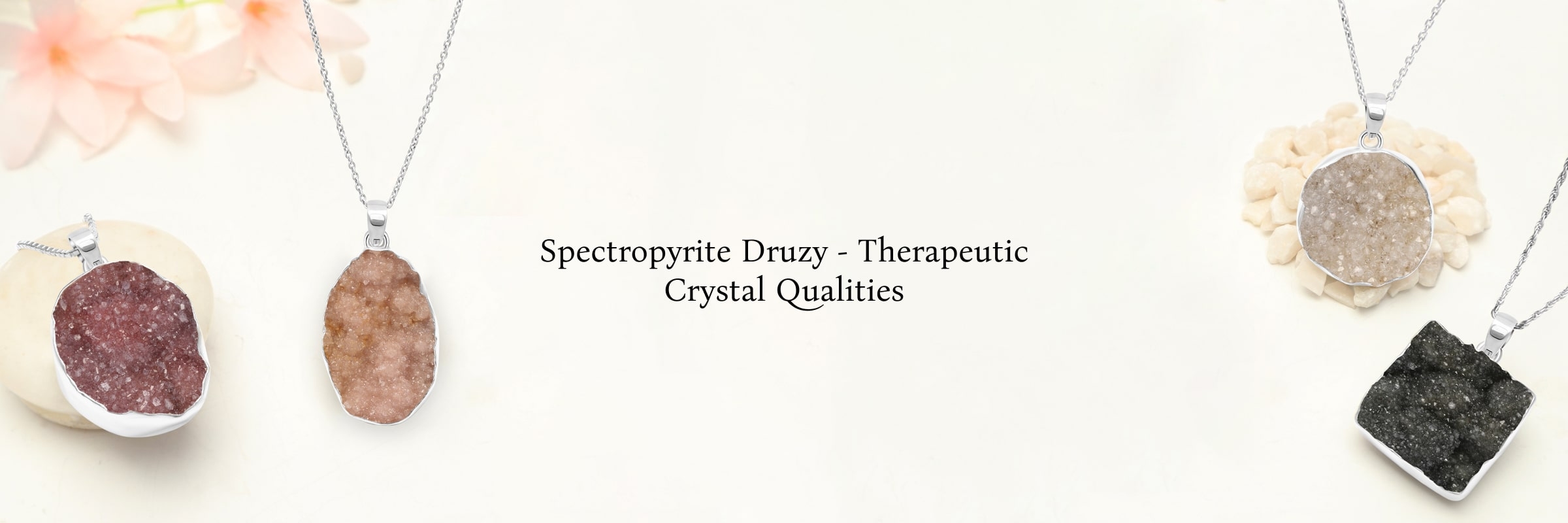The image is a detailed photograph, possibly an advertisement, showcasing four distinctive mineral pendants against a cream-colored background. The pendants, suspended from silver chains, display an array of therapeutic crystal qualities. Each pendant resembles a geode cut open to reveal intricate crystal interiors. The crystals exhibit a range of colors including dark pink, maroon, white, and black. 

The pendant on the far left is roundish with a dark pink, almost maroon hue, resembling an amethyst. Next to it, an oval-shaped pendant reveals a light-translucent white crystal interior. The third pendant showcases a white crystal inside what appears to be either a slice or a hemisphere. The final pendant on the right is square, with a striking black crystalline interior. 

In the upper left corner of the image, two delicate pink flowers embellish the scene, adding a touch of nature and softness. Additionally, two of the pendants rest on another rock, giving a natural, grounded feel, while one pendant appears to float and another lies on its side.

Centered on the image is elegant text in a fancy serif font that reads "Spectropyrite Druzy - Therapeutic Crystal Qualities," though another obscured word follows. The composition is minimalistic, emphasizing the pendants' natural beauty and the serene effect of the therapeutic crystals.